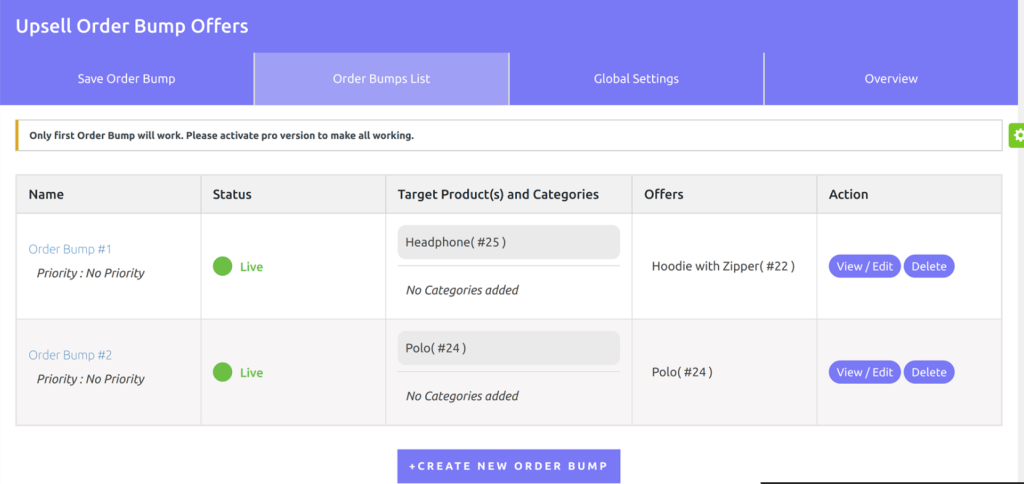This is a screenshot of a website interface designed for managing upsell order bump offers. The top of the screen features a blue navigation bar segmented into four parts by vertical lines, each labeled in white font: "Save," "Order Bump Lists," "Global Settings," and "Overview." The "Order Bump Lists" section is currently highlighted.

Beneath the navigation bar, a prominent notification box stretches across the page. It displays the message: "Only first order bump will work. Please activate pro version to make all workings," accompanied by a green gear icon on the far right.

The main content area is divided into columns labeled "Name," "Status," "Target Products and Categories," "Offers," and "Actions." The first row lists an order bump named "Order Bump Number 1" with no assigned priority. The "Status" column shows a green circle indicating the offer is live. The "Target Products and Categories" column contains "Headphones (£25)" with no categories added. The "Offers" column lists "Hoodie with Zipper (£222)." Finally, the "Actions" column provides options to "View," "Edit," or "Delete" the entry.